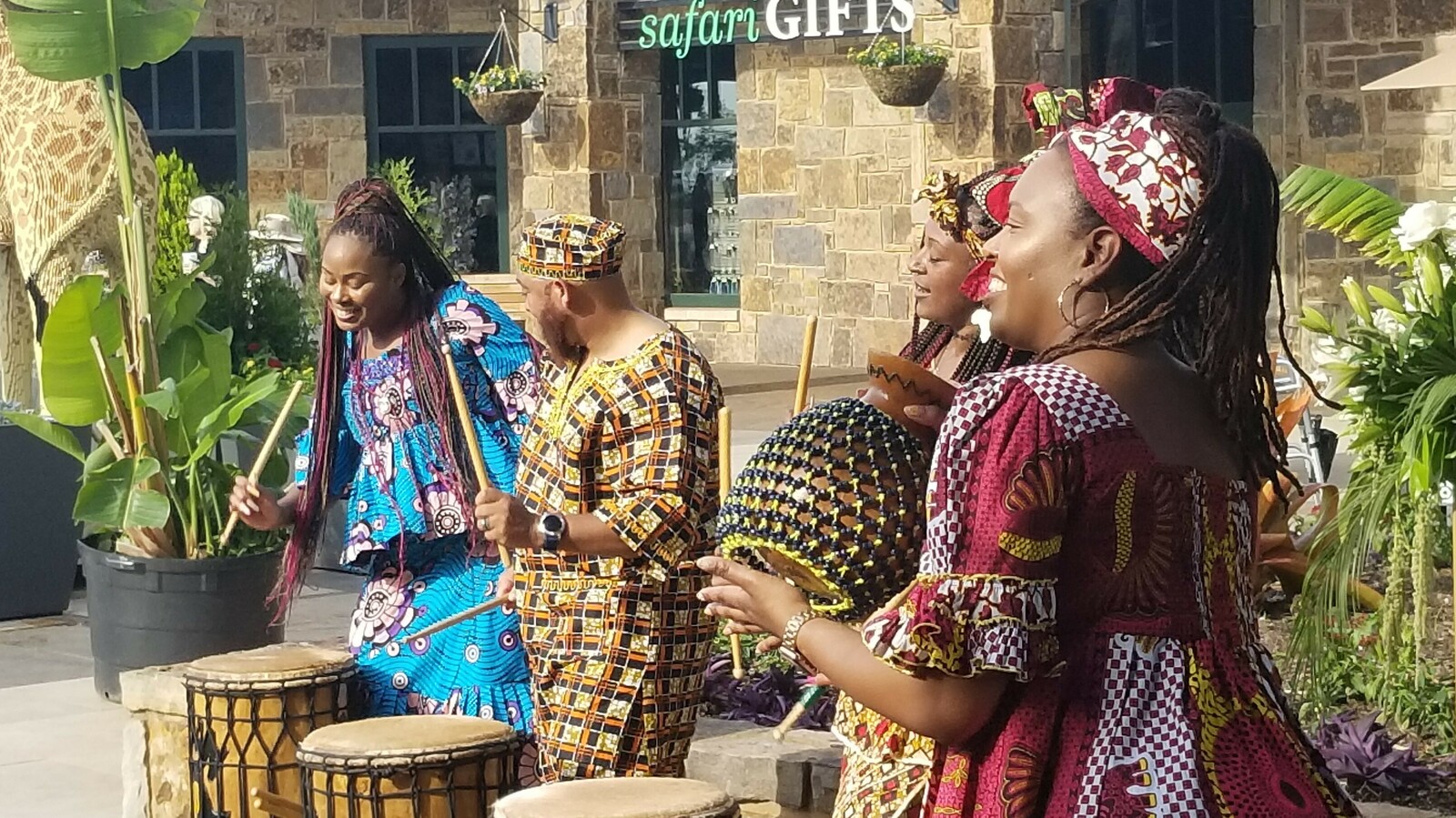The image depicts four African musicians standing outside a brick-walled building adorned with a sign reading "Safari Gifts." The storefront features large, leafy green plants on either side, resembling elephant ear plants. From left to right, we see three women and one man, each playing traditional instruments. 

The woman on the far right, a Black woman, is dressed in a vibrant red patchwork dress and matching headband, shaking an instrument that resembles a large shaker. Next to her is another woman whose face is visible, wearing a headpiece and possibly playing an unidentified instrument. The man adjacent to her sports a striking yellow and black tribal outfit with a matching hat and a prominent metal wristwatch, holding drumsticks for the bongo drums in front of him. The woman on the far left, wearing a bright blue African-style dress that covers her from neck to toe, has long braids and is also holding drumsticks.

In the background, the signage "Safari Gifts" is prominently displayed above windows, hinting at a thematic entrance, possibly to a safari attraction, and a statue of a giraffe can be faintly seen. This colorful and lively scene captures the essence of an African musical performance, set against the rich backdrop of cultural motifs and vibrant attire.